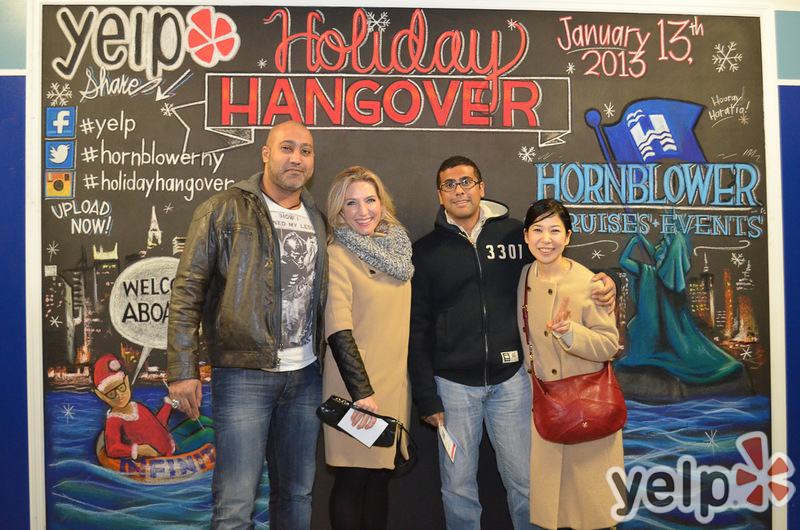In the vibrant setting of a mural marked "Holiday Hangover January 13, 2013," emblazoned with various hashtags, four individuals pose closely together, arms around each other, exuding camaraderie. The mural, rich with detail, features a whimsical city scene with an elf floating on an inner tube in water, and prominently displays "Hornblower Cruise Events."

From left to right, the first person is a bald man dressed in a brown jacket, white t-shirt, and blue jeans. Next, a blonde woman wears a brown jacket with black accents and a gray scarf, clutching a black purse. The third individual, a man with glasses, is attired in a black sweatshirt and blue jeans. Finally, a woman in a beige jacket and red purse flashes a peace sign towards the camera.

The image, a Yelp publication indicated by its logo on the bottom right corner, also features social media icons and venue information subtly integrated into the mural's design. The top left corner of the mural displays "share" next to a snowflake, alongside icons for Facebook, Twitter, and Instagram, while the Statue of Liberty holding a flag is depicted toward the bottom. This lively and detailed backdrop perfectly complements the joyful and close-knit group.